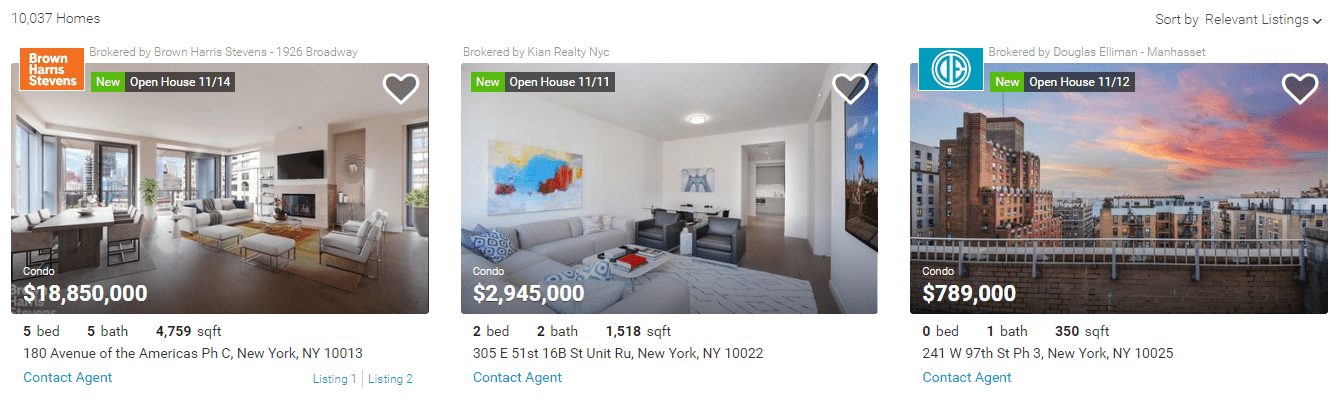A detailed screenshot displays a real estate listing for houses and condos for sale. The upper left corner indicates that there are 10,037 homes available. Three distinct condos are shown in the main section of the image with their details specified.

The first listing is highlighted with an orange rectangle labeled "Brown Harris Stevens," signifying the company managing the sale. A "NEW OPEN HOUSE 11-14" notice is also displayed. The image reveals a modern, aesthetically pleasing condo with white walls, white furniture, and large glass windows. This property is priced at $18,850,000, boasting five bedrooms and five bathrooms. It is located in New York City. Each listing features a small gray heart with a white border in the upper right corner.

The second listing, brokered by "Key and Realty," shows a cozy living room with an L-shaped sofa, white walls, black armchairs, and a gray rug. This condo is listed for $2,945,000 and offers two bedrooms, two bathrooms, and spans 1,518 square feet. It is also situated in New York City.

The third listing displays an exterior shot of some buildings under a sky with clouds. This condo, brokered by "Douglas Elliman Manhasset," is priced at $789,000 and has zero bedrooms, one bathroom, and a total area of 350 square feet. It is, too, based in New York City.

Below each property image, there is a blue link stating "Contact Agent," inviting potential buyers to reach out for more information.